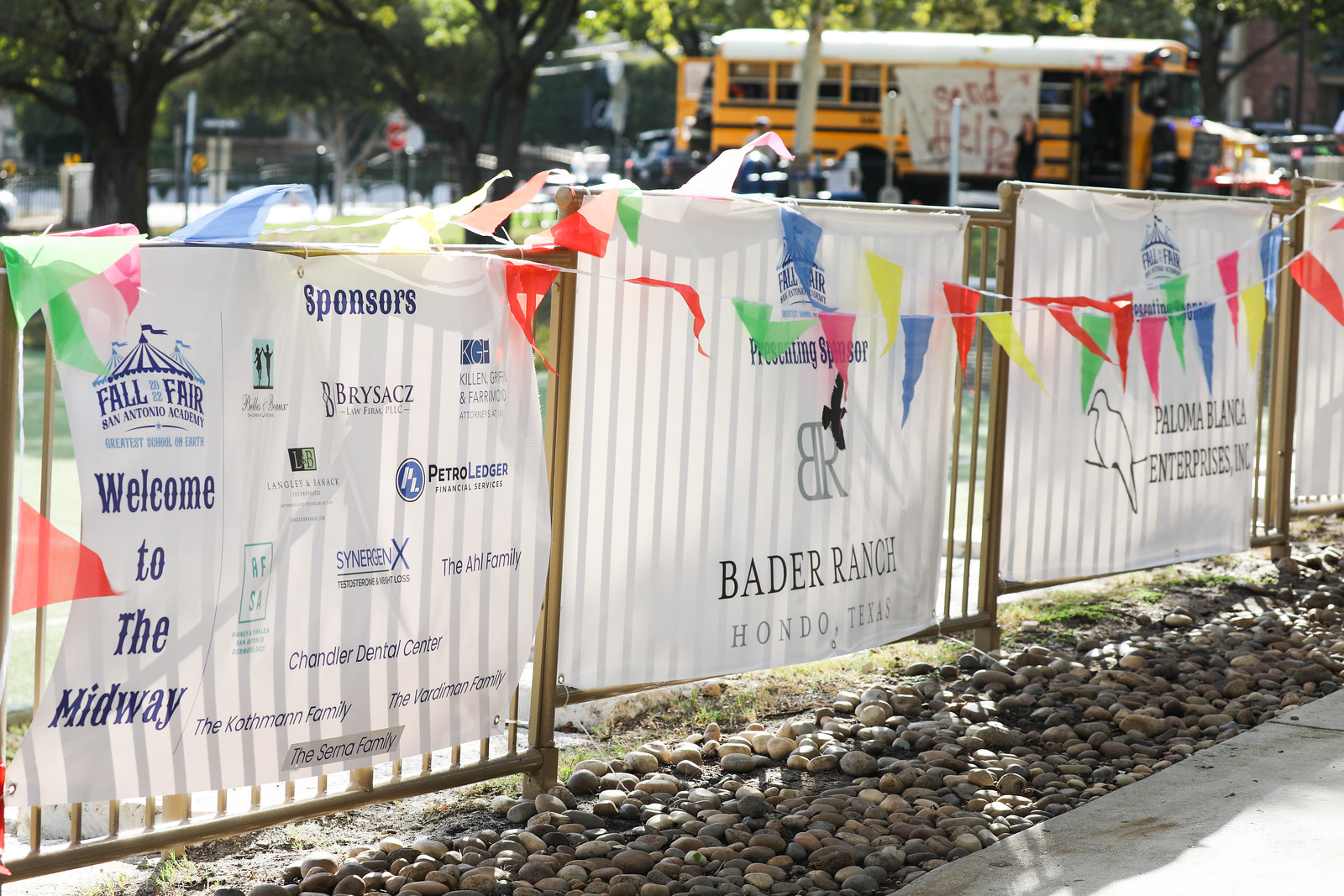The image depicts a lively outdoor setting centered around a decorative fence adorned with colorful, rainbow-like pennant banners. Below the banners are multiple advertisement signs promoting the Fall Fair at San Antonio Academy, with slogans such as "Welcome to the Midway" and "Greatest School on Earth," listing sponsors including Bader Ranch from Hondo, Texas, and Paloma Blanca Enterprises Inc., as well as others like Petroledger, Synergex, and Chandler Dental Center. The fence stands above a base of larger gravel, next to a sidewalk. In the background, large school buses are visible, one with a prominent red banner reading "Send Help," which adds a curious and possibly humorous element. The scene also features lush trees, suggesting a park-like environment, contributing to the festive atmosphere.